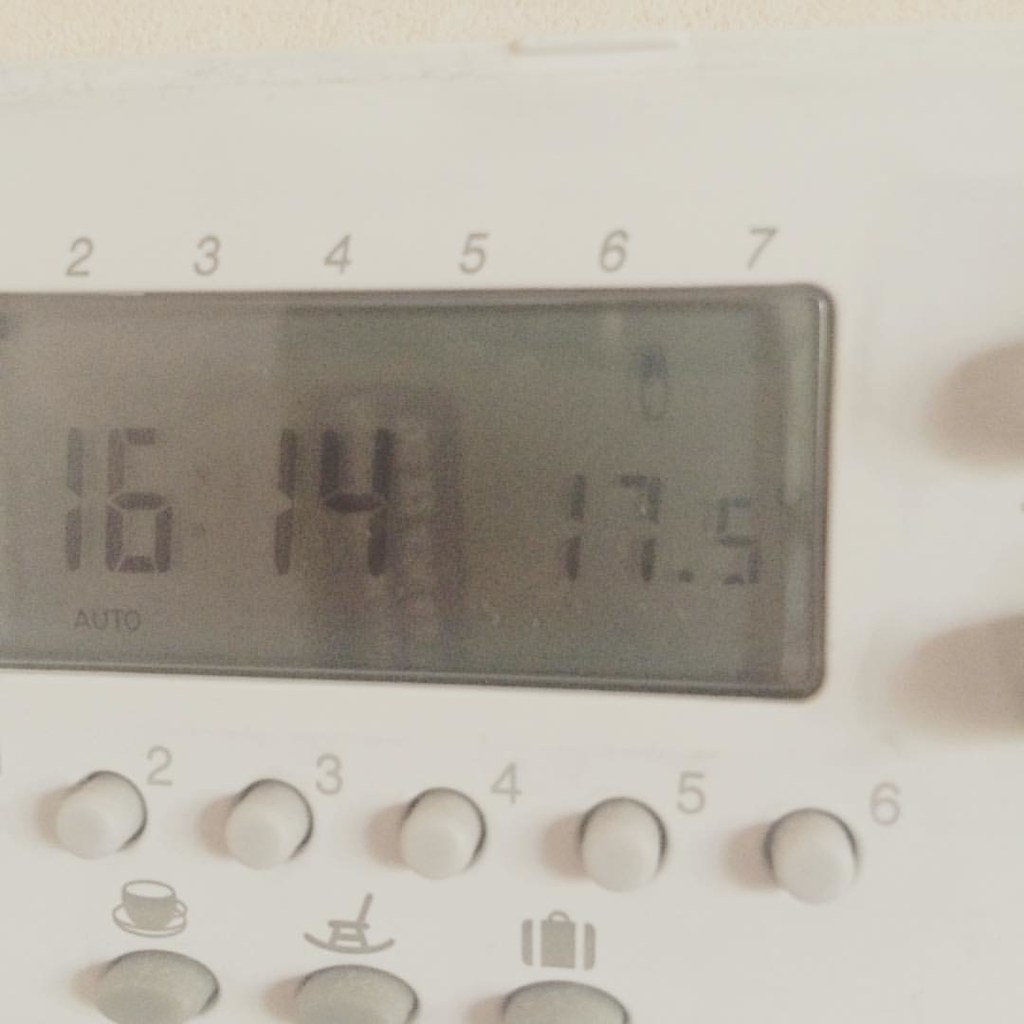The image features a close-up of a device that appears to be either an alarm clock or a thermostat. Centrally positioned on the device is a digital screen displaying the numbers 16, 14, and 17.5, along with the word "auto." Surrounding the screen are clearly labeled buttons: numbers 2 through 7 are listed above, and numbers 2 through 6 are listed below. Below these buttons, there are three additional buttons, each displaying distinct icons: a coffee cup, a rocking chair, and a suitcase. The background of the image reveals a white wall, though the focus remains mainly on the device. This device likely serves to modify settings, indicated by its various buttons and screen.